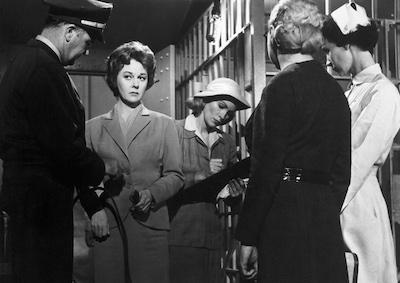This evocative black-and-white photograph appears to be a still from an old movie, capturing a tense and atmospheric moment possibly set on a movie set. In the foreground, to the far left, stands a man in a police uniform complete with a cap, facing right and looking down, perhaps in a moment of admonishment or serious conversation. His stance and uniform signal authority. Next to him is a distressed-looking woman with short dark hair, wearing a neatly tailored pantsuit. She is gazing off to the side at the policeman, her expression suggesting nervousness or unease. 

To the right of this woman, another woman is absorbed in writing on a clipboard she holds. This woman is wearing a hat and a light-colored blouse under a darker dress, her focus entirely on her task. Behind her, partially obscured, is another female figure dressed in a long black coat, seen from behind. At the far right stands a woman in a white nurse's uniform, complete with a nurse's cap and her hair pinned up. She has her head slightly bowed, adding to the somber or serious mood of the scene. The background features metal bars, implying they are positioned in front of a jail cell, which further intensifies the dramatic atmosphere captured in this image.